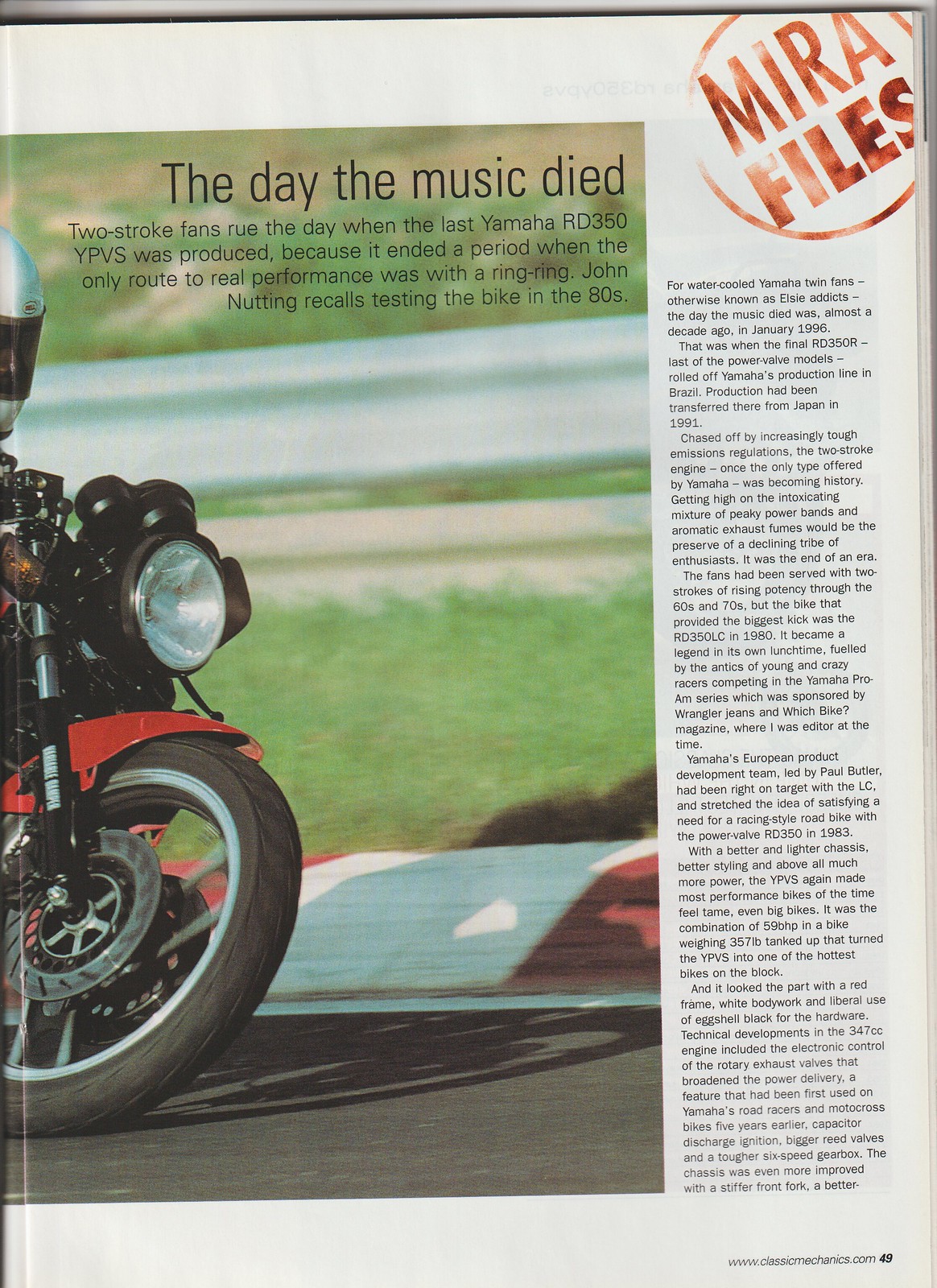The magazine ad captures a nostalgic moment for motorcycle enthusiasts, prominently featuring a vivid photograph of a Yamaha RD350 YPVS. The image reveals the front wheel, red fender, headlight, and a portion of a white helmet, set against a green, grass-like background, suggesting a racetrack environment. At the top, bold black text announces, "The day the music died," referencing the lament of two-stroke fans for the discontinuation of the iconic RD350 YPVS. The ad speaks to the era when two-stroke engines were the epitome of performance, providing unmatched power and a distinctive sound—recalled with fondness by John Nutting, who tested the bike in the 80s.

The right side of the page presents a dense column of text, chronicling the history and impact of the RD350 YPVS. It mourns the end of an era for water-cooled Yamaha twin fans, also known as Elsie Attics, specifically noting January 1996, when the final RD350R was produced in Brazil. This transition marked the beginning of tougher emissions regulations and the gradual phasing out of two-stroke engines. The narrative celebrates the evolution of Yamaha's two-stroke engines, highlighting the RD350LC's legendary status in 1980 and its significant role in the Yamaha Pro-Am Series. It details the innovative advancements in the RD350's 347cc engine, such as the electronic control of rotary exhaust valves and capacitor discharge ignition.

The ad is part of page 49, as noted in the bottom right corner, alongside a somewhat illegible website URL, likely www.classicmechanics.com. Subtle yet informative, the layout and imagery collectively honor the storied past of Yamaha's RD350 YPVS, a motorcycle that defined an era for performance biking enthusiasts.